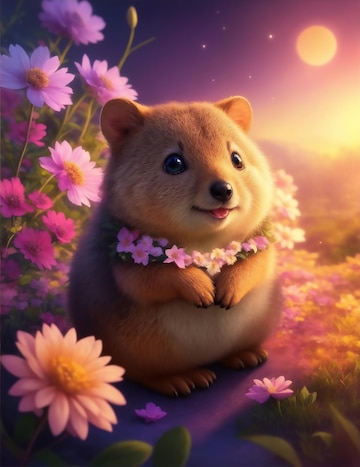This animated image showcases an adorable small creature, reminiscent of a gopher or gerbil, adorned with a garland of pink flowers around its neck. The furry mammal, characterized by its soft brown fur, rounded ears, and shiny, dark round eyes, has a cute expression with its black nose and a tiny pink tongue sticking out from its small mouth. The critter stands upright on its hind feet, with its front paws held in front like hands, in a picturesque nighttime setting. The background features a stunning night sky with a full, orangish moon in the upper right corner and several stars to the left, casting a moonlit glow over the scene. Behind the creature is an assortment of beautiful wildflowers, including some pink cosmos and other pink varieties, with additional green leaves enhancing the natural ambiance. In the bottom left corner of the image, there's a prominent pink flower with three rows of pointed petals and a yellow center, adding to the delightful and whimsical atmosphere.